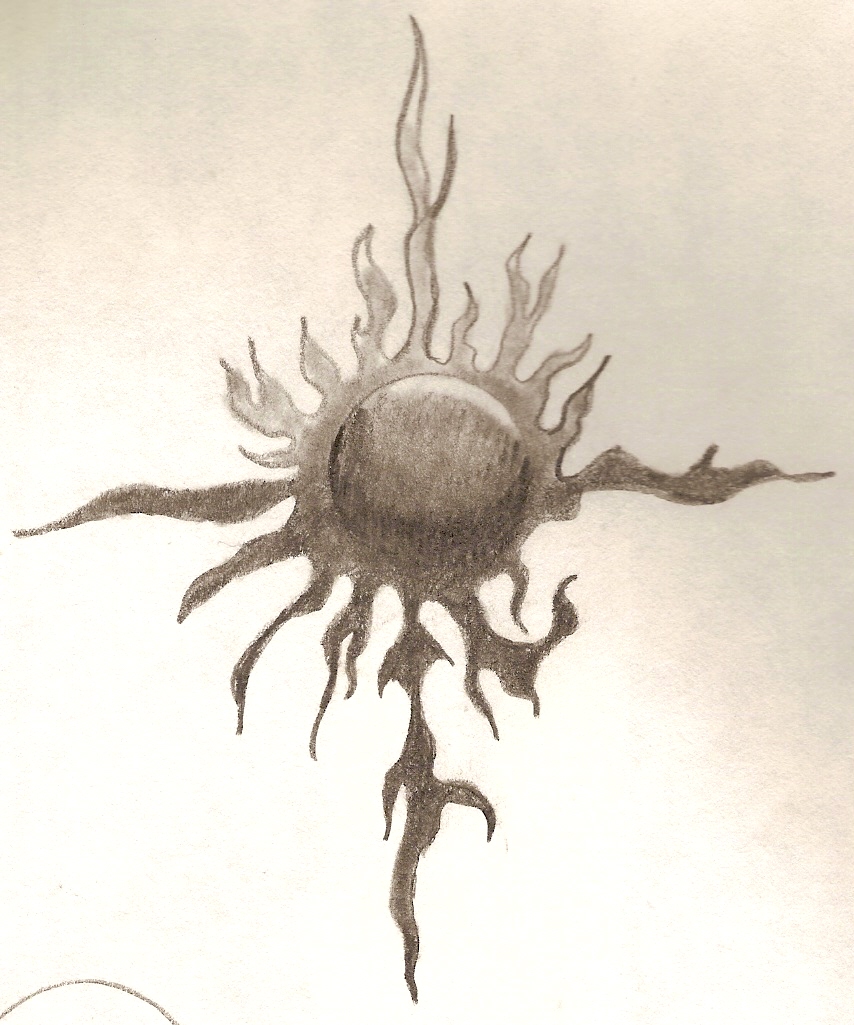This image is a detailed pencil drawing on plain white paper, somewhat resembling a sketch pad or canvas. The drawing features a central circular object, reminiscent of a fiery sphere or sun. This central disc is shaded progressively, appearing lighter at the top and gradually darkening towards the bottom, with no distinct line of demarcation.

Surrounding the circle are numerous flame-like designs that radiate outward in every direction. These flames have an organic and wavy appearance, with four prominent flames extending farther from the circle at the positions corresponding to 12, 3, 6, and 9 on a clock face. Other shorter flames fill the spaces in between these longer ones. The flames are shaded similarly to the central circle, with the tips being lighter and progressively darkening towards the base, providing a gradient effect across the drawing.

In the lower left corner, there is a curved line resembling a half-moon shape, facing downwards, adding an additional element to the artwork. The overall image combines these elements into a cohesive and dynamic hand-drawn design that captures the eye with its intricate shading and flowing forms.